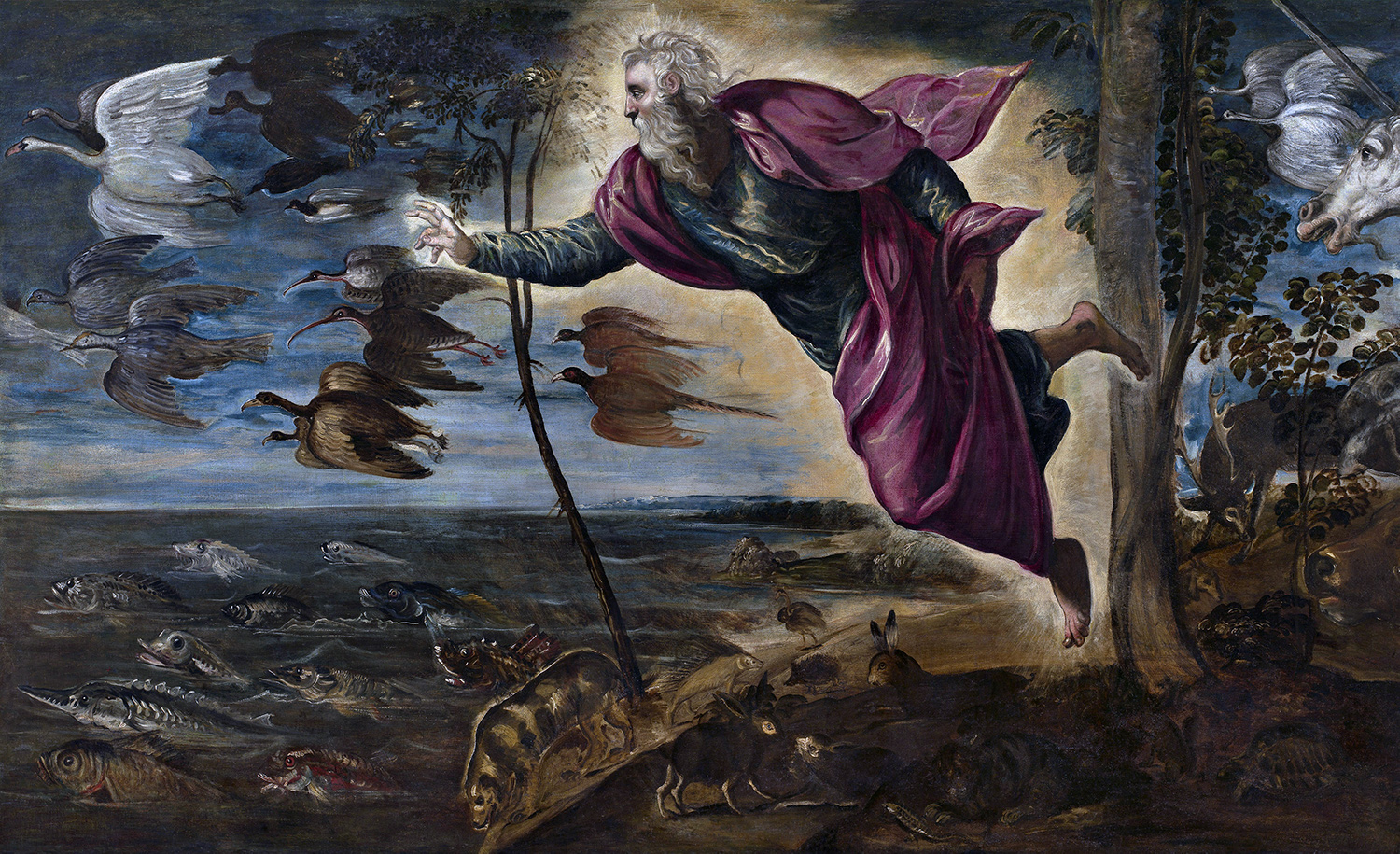The image depicts an enchanting biblical painting set against a dark night sky. The central figure, an older man with long gray hair and a flowing gray beard, is surrounded by a glowing halo effect and appears to be floating in mid-air. He is dressed in a billowing purple robe that extends dramatically behind him over a blue or black garment, and he is barefoot. His right arm is outstretched, as if commanding the elements or the creatures around him.

Surrounding the figure are various animals. Below him on the ground, partially camouflaged by the brown earth, is a rabbit. In the air to the left, various species of birds, resembling ducks and geese with white leading the flock, appear to be flying, their wings spread wide. There is also a white horse’s head, mouth slightly open, peering from the upper right corner. Behind the man stands a sparse tree with a thin trunk, alongside another with a thicker trunk and small leaves.

Below the floating figure, a murky river teems with different species of fish, all directed to the left, including what appears to be a sawfish, a swordfish, and perhaps others with bulging eyes that give them an eerie appearance. Additionally, at the bottom left of the river scene, a mollusk can be seen. This mystical painting, likely a nocturnal depiction, blends elements of nature and the supernatural, creating a rich, detailed tableau that evokes a sense of divinity and wonder.